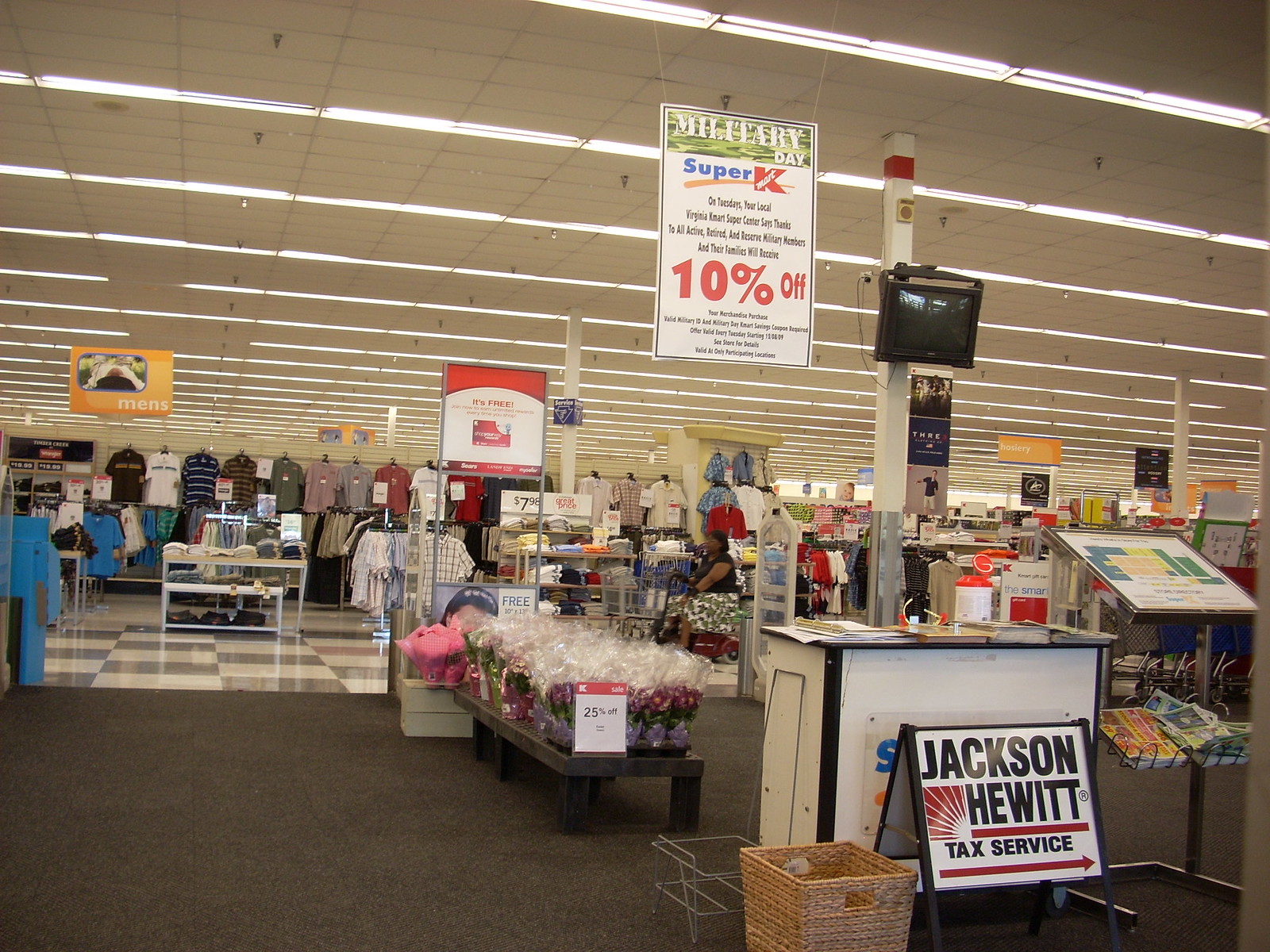This photograph depicts the interior of a Kmart store, specifically highlighting the menswear section in the background. A prominent banner hangs from the ceiling reading, "Military Day Super Kmart 10% off." In the foreground, there's a sandwich board style sign for "Jackson Hewitt Tax Service" with a red arrow pointing to the right. Behind this sign, there's a small white station with an old-fashioned square black television mounted above it, possibly for security purposes. Nearby, a wicker basket sits on the floor. Additionally, a rectangular table displaying discounted, cellophane-wrapped flowers is visible, marked down by 25%. The floor transitions from brown carpet in the foreground to white and gray tiles in the background. The well-lit ceiling features fluorescent light fixtures extending throughout the store. The menswear section itself is filled with a variety of shirt patterns including black, white, white and blue stripes, green, and gray, displayed on numerous clothing racks and shelves.